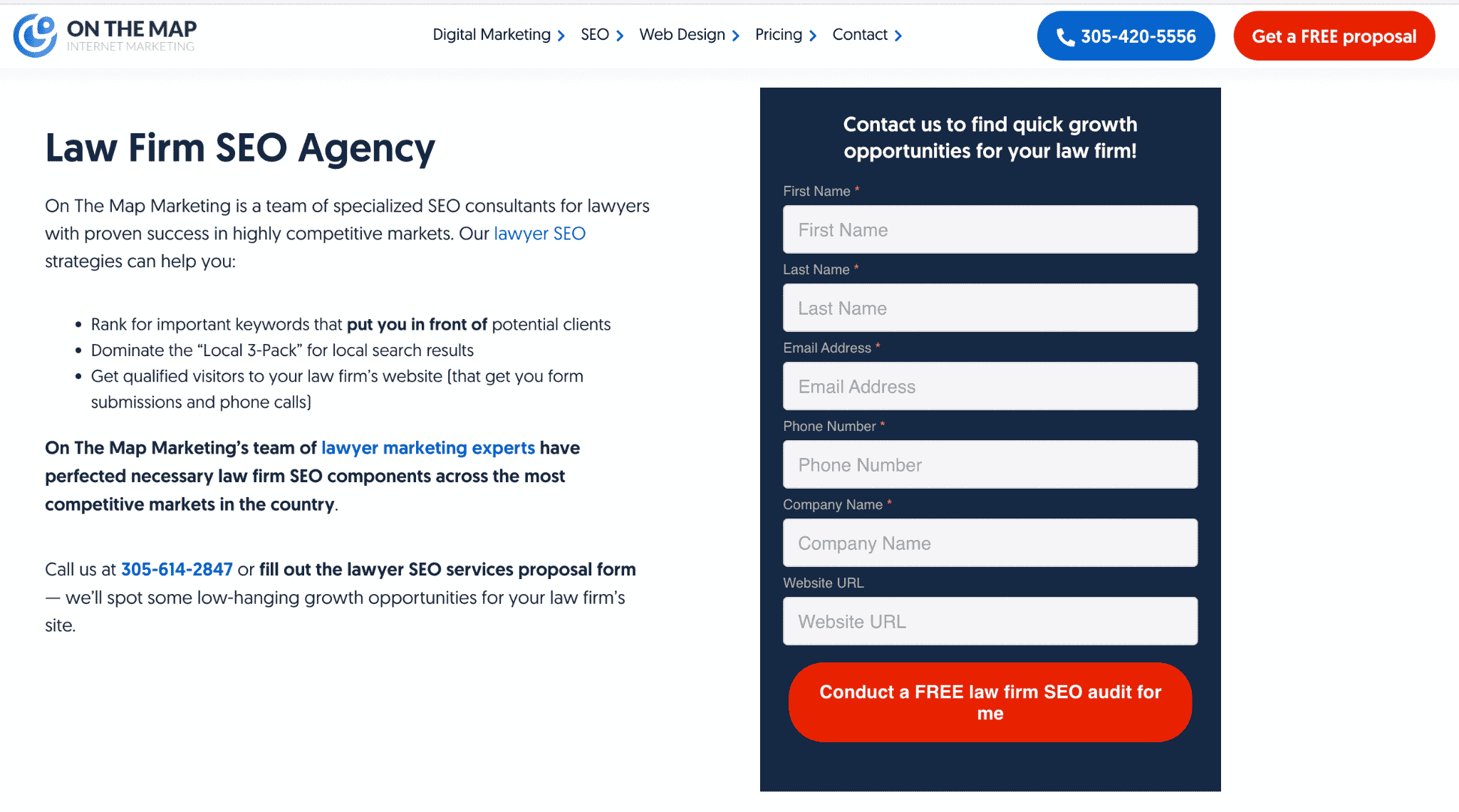The image showcases a website interface centered on a map theme. In the upper left corner, there's a blue and white symbol, followed by the text "On the Map." Right next to it, the header includes navigation links: "Digital Marketing," "SEO," "Web Design," "Pricing," and "Contact." In the upper right corner, there's a blue phone icon with a phone number next to it. Adjacent to this is a red bubble with white text reading, "Get a Free Proposal."

Beneath this top section, there's a call-to-action area on the right encouraging visitors to "Contact us to find quick growth opportunities for your law firm." This includes input fields for first and last name, email address, phone number, company name, and website URL. Below these fields, a button prompts users to "Conduct a Free Law Firm SEO Audit for Me."

On the left side, bold text reads "Law Firm SEO Agency," accompanied by detailed information about their services. There are also clickable sections with hyperlinks and a phone number displayed in the bottom left corner for further contact.